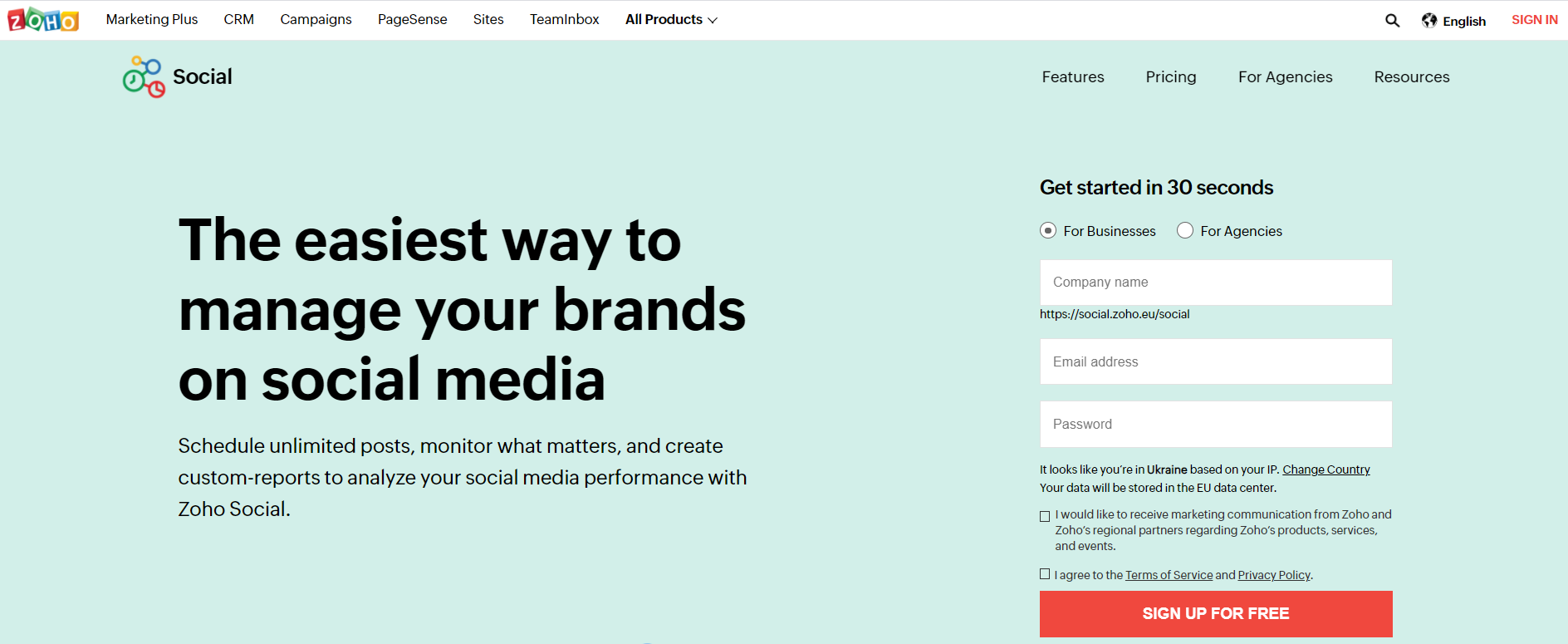**Descriptive Caption:**

This screenshot, captured from the Zoho website in a desktop or laptop view, showcases the user interface and options available for Zoho Social. In the upper left corner, the Zoho logo is prominently displayed beside a navigation menu listing several products: Marketing Plus, CRM, Campaigns, PageSense, Sites, TeamInbox, and an option to view all products. Below the navigation menu, the headline reads, "The easiest ways to manage your brands on social media," followed by a brief description that emphasizes the platform's capabilities such as scheduling unlimited posts, monitoring relevant metrics, and creating custom reports to analyze social media performance.

On the right side of the screenshot, several tabs are visible, including Features, Pricing for Agencies, and Resources. There is a prominent call-to-action offering to "Get started in 30 seconds," with specific options tailored for either businesses or agencies. Below this, fields are available for users to input their company name, email address, and password. Additionally, a notification indicates that the user’s IP address suggests they are in Ukraine, with an option to change the country, specifying that their data will be stored in the EU data center. The layout of the image is rectangular, encapsulating all these details clearly and concisely.